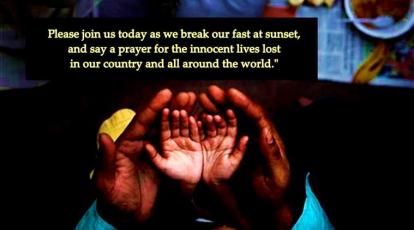A color photograph with a black background features white text at the top that reads: "Please join us today as we break our fast at sunset and say a prayer for the innocent lives lost in our country and all around the world." Below this text, a pair of large adult hands cradles a smaller set of infant or young child’s hands, both sets with African or African-American skin tones. The adult, likely a parent, wears a light blue collared shirt, visible at the edges of the hands. In the upper right corner of the image, a bowl of food references the meal to break the fast mentioned in the text. The composition of the photograph focuses solely on the hands, offering a poignant and intimate visual centered on unity and prayer.